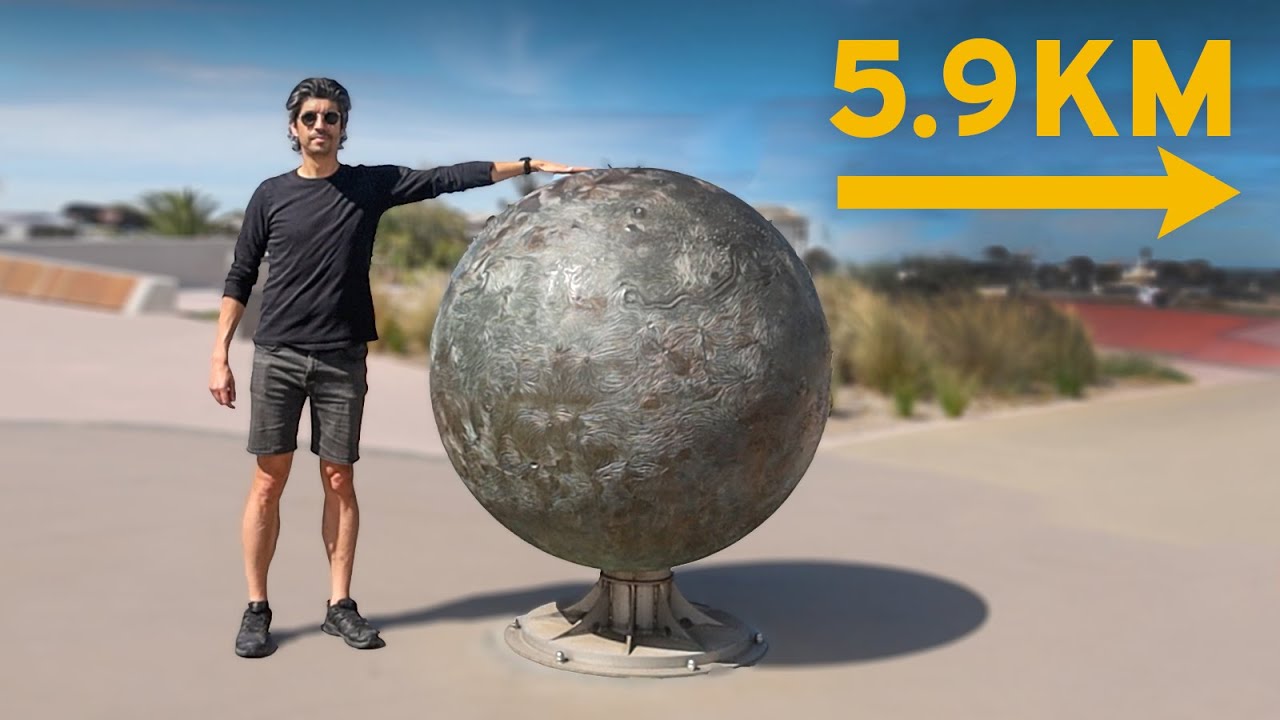In this vibrant color photograph, a bearded man with dark hair, clad in a black long-sleeve t-shirt, gray shorts, and black sneakers, stands confidently under a sunny blue sky dotted with wispy clouds. With his left hand resting on the apex of an imposing spherical structure, he appears engaged and almost contemplative. This large orb, resembling a planetary model, is crafted from a silvery-gray metal with faint light-red accents and distinct etched details. It is securely mounted on a robust pedestal, bolted into a beige concrete walkway, implying permanence and weight. Behind him, greenery and brush suggest a landscaped area, possibly in a southwestern region like Arizona. In the upper right corner of the image, a prominent yellow arrow accompanied by the text "5.9 KM" directs attention to the right. Hints of additional structures, possibly a running track, linger subtly in the backdrop, adding layers of context to this intriguing scene.